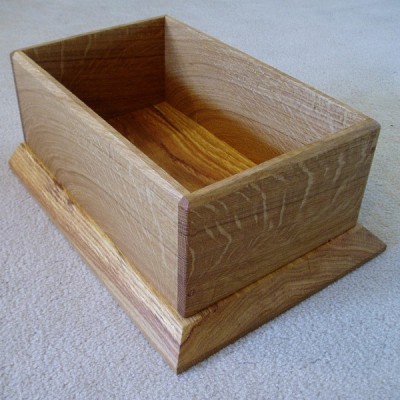The image showcases a handcrafted rectangular wooden box sitting on a clean, short white carpet. The box, constructed from light brown wood with noticeable grain patterns, appears to lack a lid, resembling a chest or catch-all. Both the darker wooden base and the trapezoidal frame suggest it was recently built. Its muted neutral tones match the surrounding gray background, giving an overall impression of a simple yet meticulously crafted wooden item. The sides of the box have rough textures, possibly due to scratches or an unfinished wood grain, and are slightly whitewashed, contrasting with the darker base.